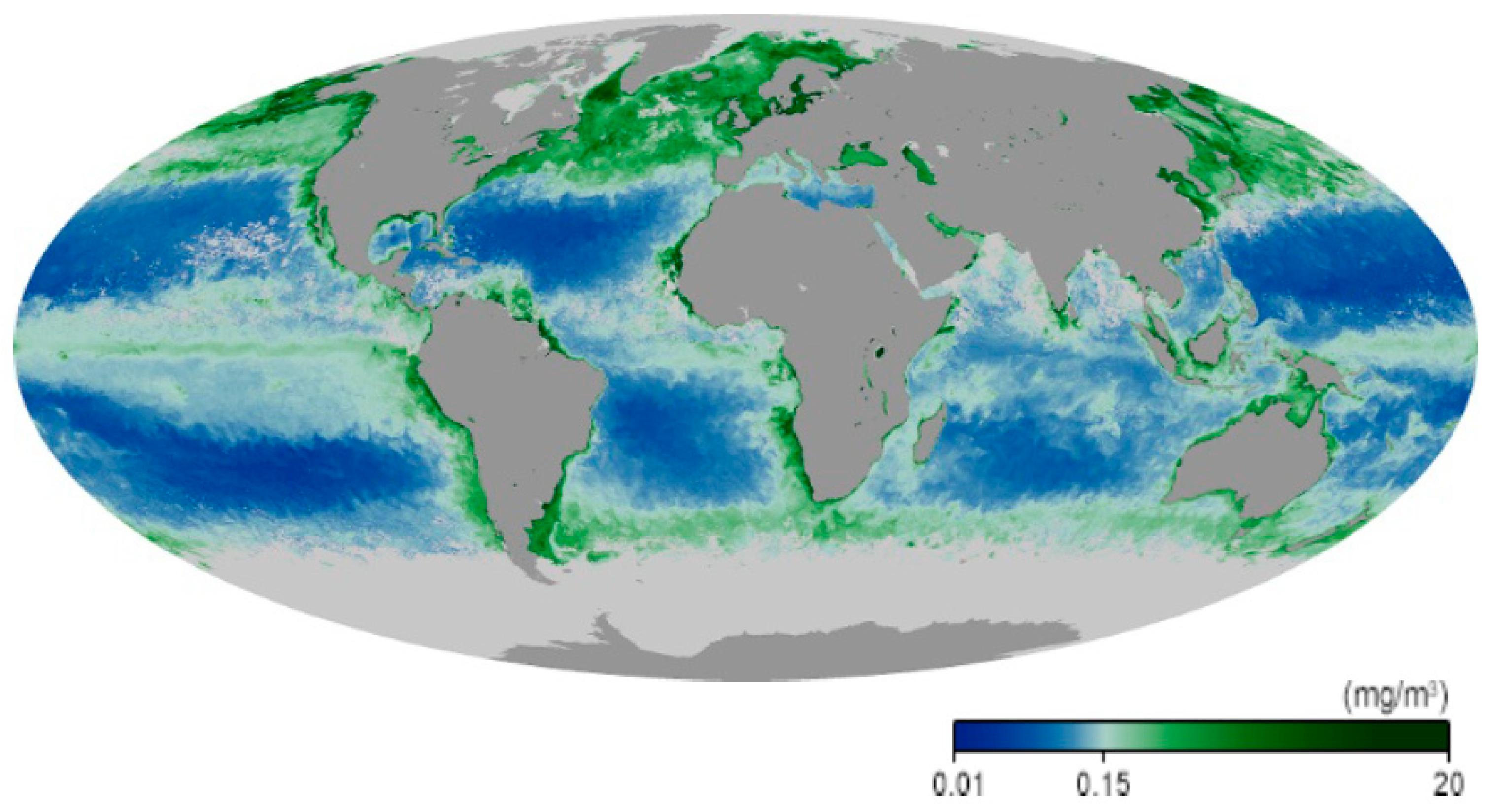This image is a digital infographic depicting a map of the Earth in a squished oval shape, possibly resembling a Makita projection or another type of flattened map demonstration. The continents, including North America, South America, Africa, Europe, Asia, Australia, and Antarctica, are shown in gray, while the oceans predominantly feature blue and green hues. The green areas are prominently depicted between North America and Greenland, as well as above Europe, around Alaska, and near other continental coastlines. The map is presented against a white background, with a color scale below it representing measurements in milligrams per cubic meter (mg/m³). The scale ranges from dark blue, indicating values of 0.01, to dark green, representing values of up to 20, with an intermediate white section denoting 0.15.